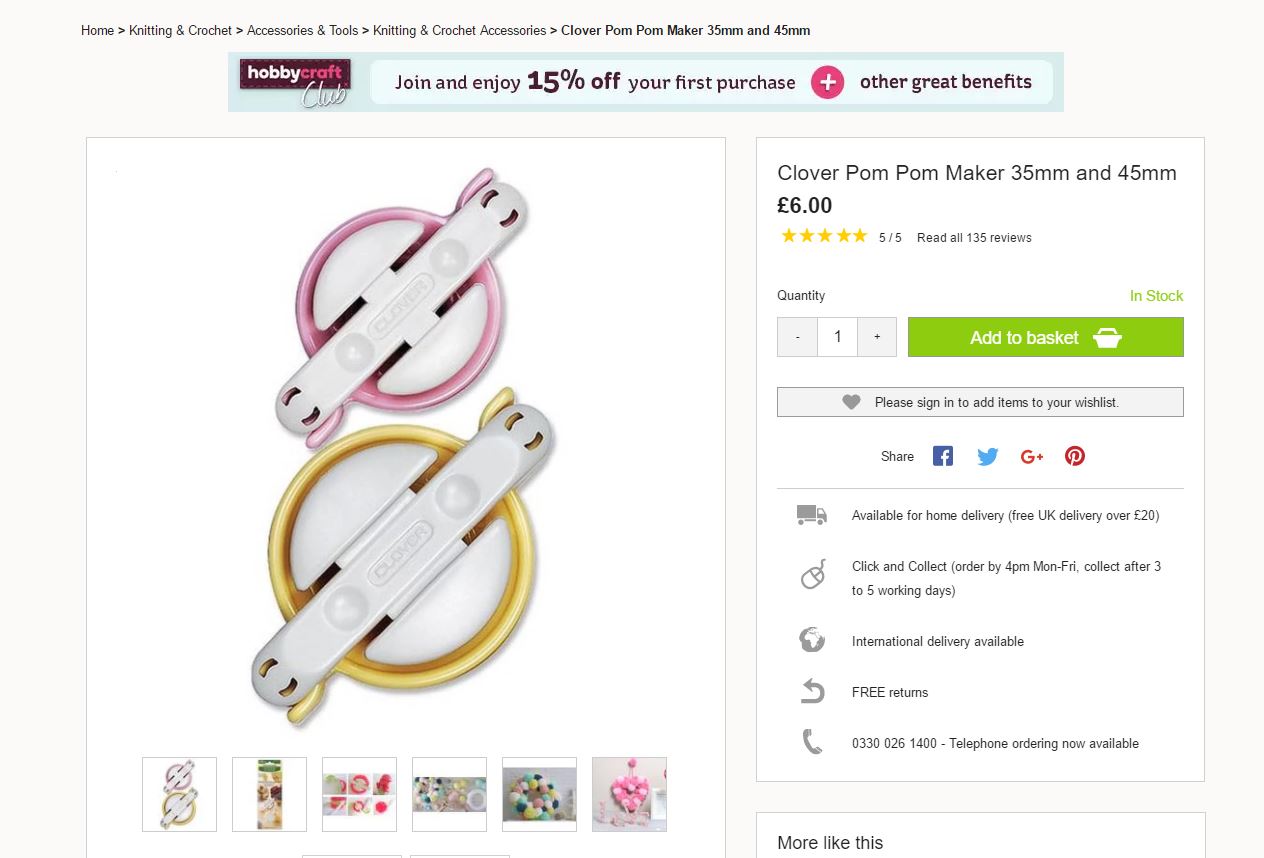A detailed caption for the described image could be:

"Screen capture of the Hobby Crafts Club website, featuring a prominent logo at the top. The site offers a special promotion: 'Join and enjoy 15% off your first purchase.' The main product displayed is the 'Clover Pom-Pom Maker (35mm and 45mm),' priced at £6 for the set. The image showcases two pom-pom makers – the larger and smaller rings are designed to help create uniform pom-poms by winding yarn around the rings and spinning the inner device. Smaller thumbnail images beneath the main product offer glimpses of finished pom-poms, though their details are hard to discern due to their size. An ordering section allows users to select the quantity to add to their basket, which is not visible in the screen capture, possibly because no items have been added to the cart yet."